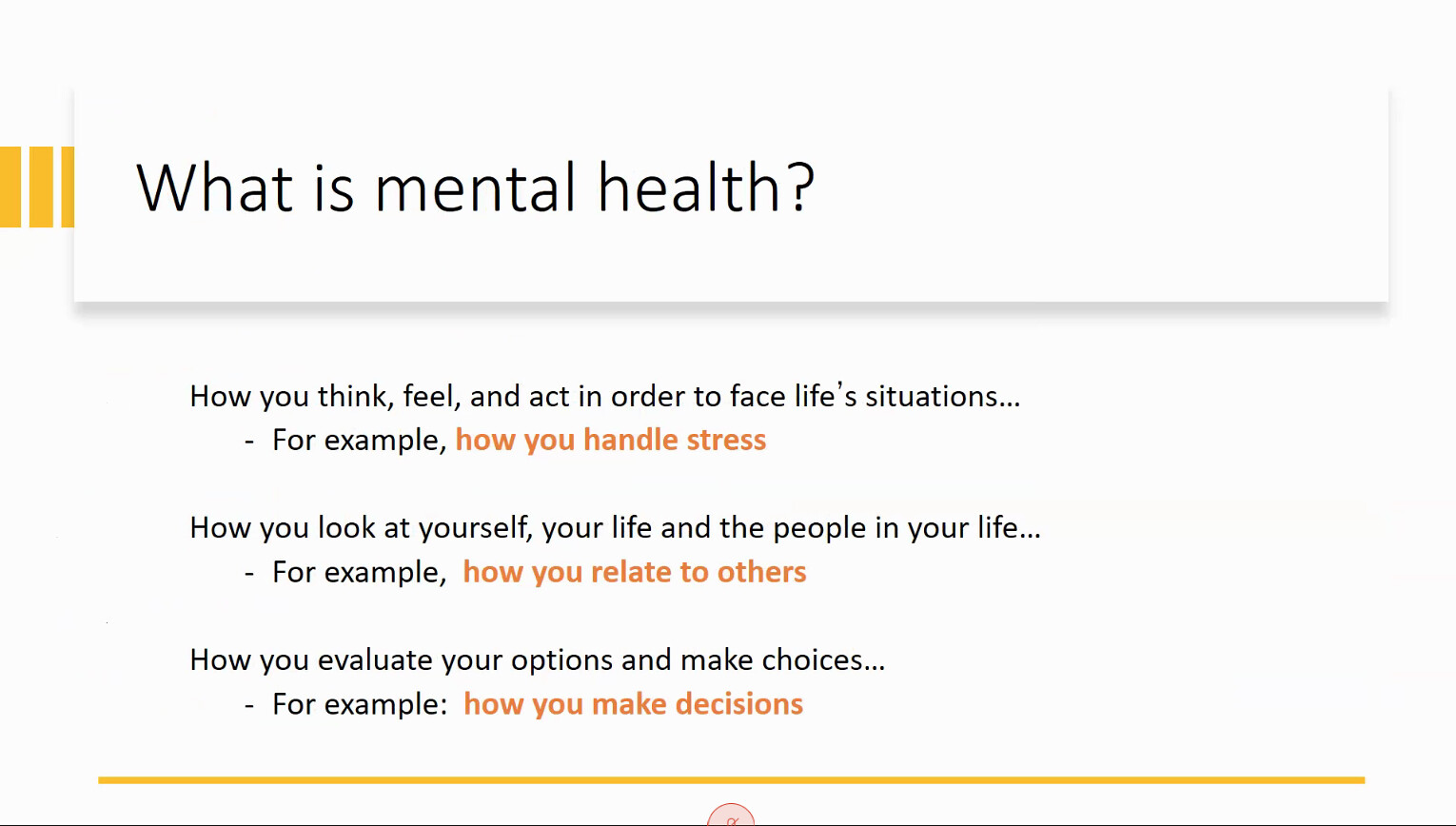The image features a clean, white background resembling a PowerPoint slide or a section from a textbook. At the top, there are small yellow rectangular symbols, and central to the page, the title reads in black text, "What is mental health?" followed by a question mark. Below this title, a thin, gray stripe spans across the page, underneath which the text elaborates on mental health.

The explanation is broken down into several lines and uses different font colors to emphasize distinct aspects. The first line, in black font, reads, "How you think, feel, and act in order to face life situations." This is followed by "for example," and subsequent lines offer specific illustrations: 

- "How you handle stress" appears in orange text. 
- Another example, "How you look at yourself, your life, and the people in your life," is also in black text, followed by, "how you relate to others," in orange font.
- Further down, the line "How you evaluate your options and make choices," in black font, is followed by an orange example, "how you make decisions."

Towards the bottom of the image, there is a yellow line followed by a black stripe. The visual elements conclude with a small, pink semicircle at the bottom.